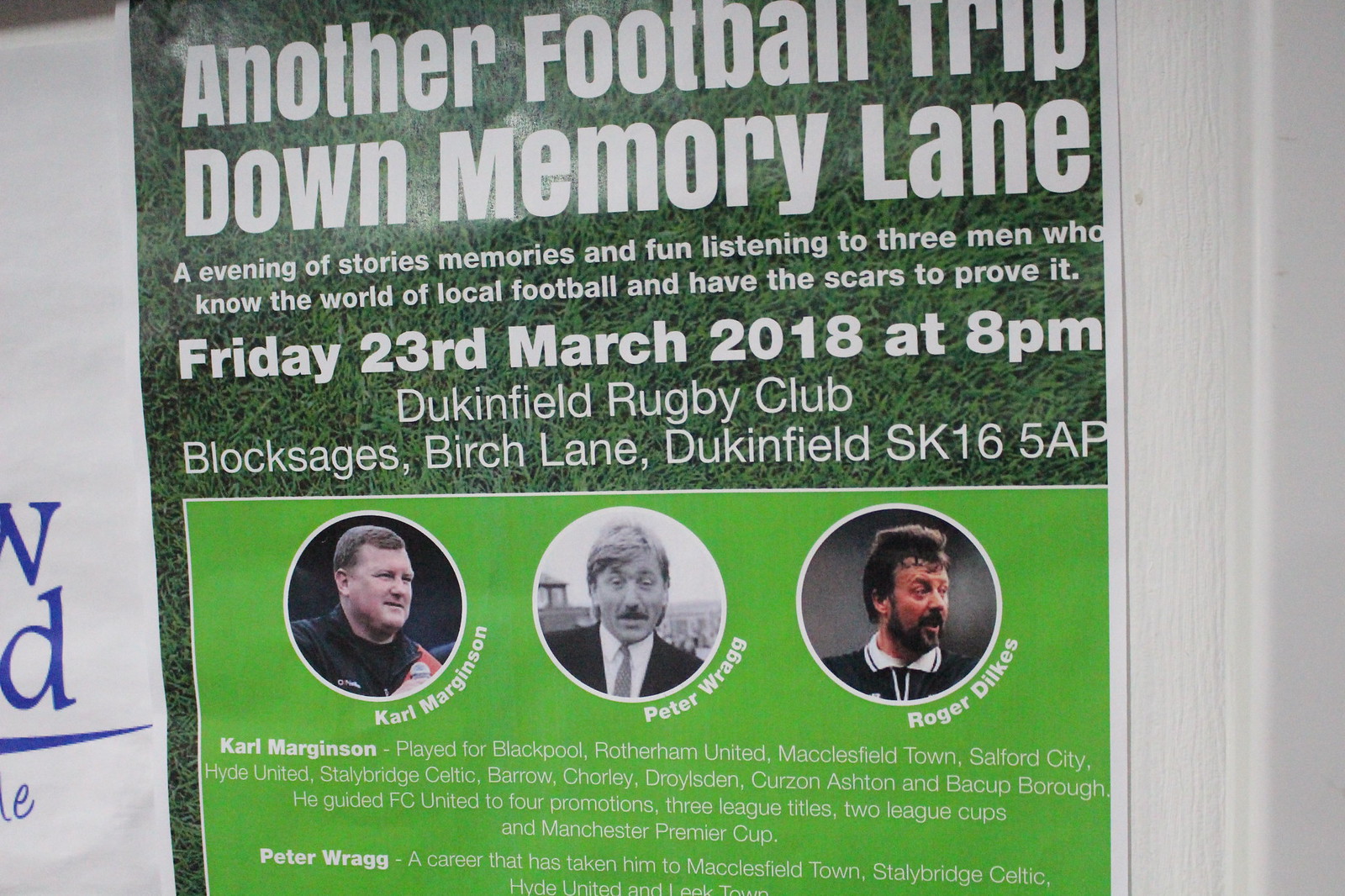This image is a poster hanging on a white wall, entitled "Another Football Trip Down Memory Lane" in white text on a green background that resembles grass, giving it the feel of a football field. Below the title, the subtitle reads, "An Evening of Stories, Memories, and Fun, Listening to Three Men Who Know the World of Local Football and Have the Scars to Prove It." The event is detailed further: "Friday, 23rd March 2018 at 8 p.m., Dukinfield Rugby Club, Black Sages, Birch Lane, Dukinfield, SK16 5AP." The poster features circular photographs of three men—Carl Marginson, Peter Wragg, and Roger Deakin—with white borders around the photos. Each man's biography, though partially cut off in the image, is displayed below their respective photos, detailing their careers and contributions to local football.